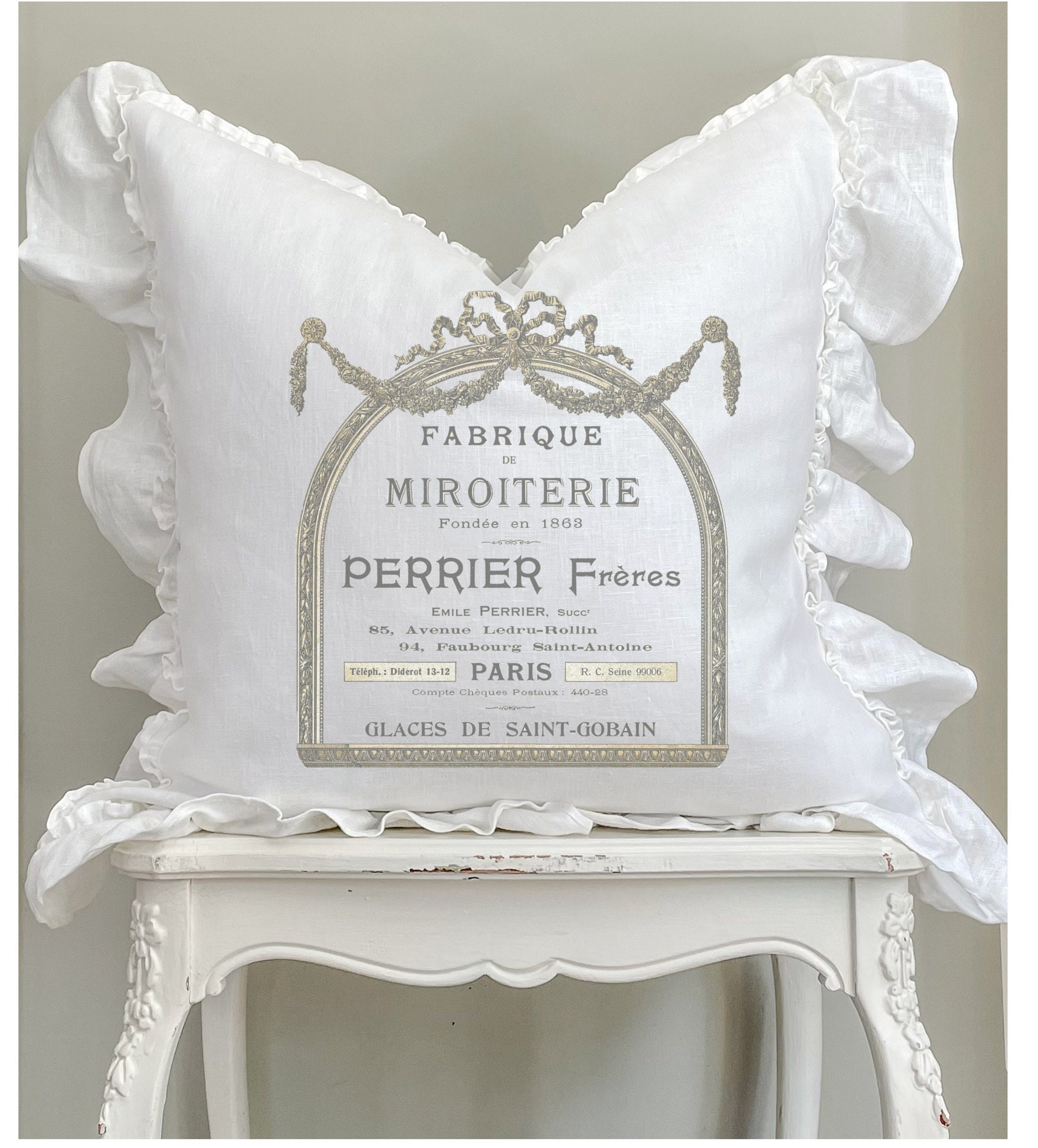The image captures an intricately detailed white pillow with silver and gray accents, displaying elegant French text and elaborate embroidery. The text includes "Fabrique de Mirotois Fondée en 1863," "Perrier Frere," "Amel Perrier," an address "85 Avenue, L'Edouardian, 94 Faubourg Saint-Antoine, Paris," and "Glace de Saint-Gobain." The pillow, shaped with a heart-like arch at the top and padded to form a V in the middle, showcases delicate white ruffles around its edges, adding to its frilly and lacy appearance. It's laid out decoratively on a small, white, distressed nightstand that features floral carvings on its front legs, all set against a white cloth backdrop.